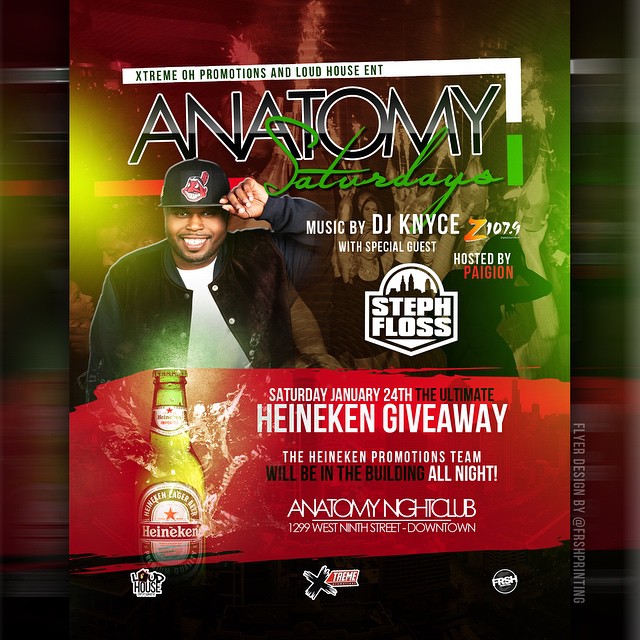This detailed flyer for Autonomy Saturdays promotes an exciting event at Autonomy Nightclub, located at 1299 West 9th Street, Downtown, on Saturday, January 24th. The evening will feature music by DJ K-Nice, with special guest Stepfloss, and will be hosted by Pagan, all under the sponsorship of Z107.9, Extreme OH Promotions, and Loud House ENT. The ultimate Heineken giveaway is a highlight, with the Heineken Promotions team present all night, evidenced by the flyer showing a Heineken bottle. Designed by FRSHPRINTING, the flyer prominently features club imagery with a DJ in the foreground and various logos at the bottom, marking it as a significant promotional event.